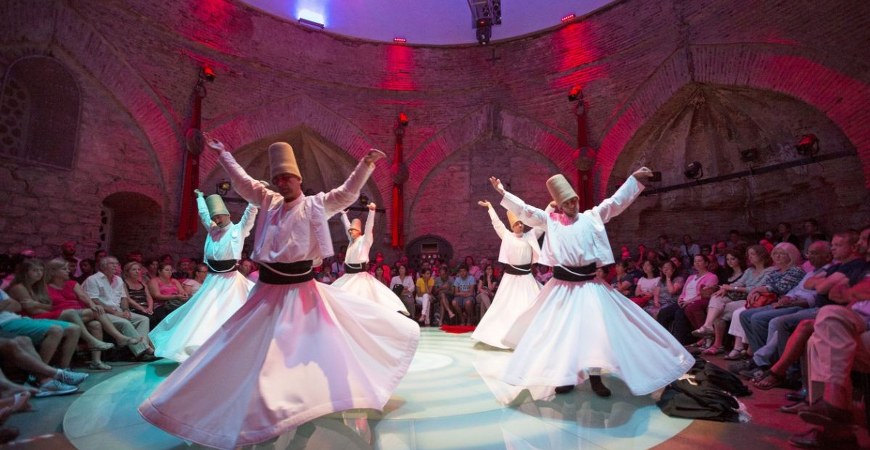In the evening light of an outdoor amphitheater that resembles a Turkish palace with vintage Mughal or Persian architectural elements, including rock and brick walls and significant wooden doors, a captivating scene is unfolding. The audience, composed of both men and women of various ages, is seated in a circular arrangement around a central, blue-colored stage, which is bathed in spotlight and rimmed with red lighting. On this stage, several dancers donning traditional Sufi costumes are performing. They wear long, white robes that flare out beautifully as they spin, black belts, and form-fitting beige hats resembling thimbles. The dancers, who appear to be white or Caucasian, hold their hands up and elegantly revolve around each other, their movements creating a mesmerizing display for the entranced audience.